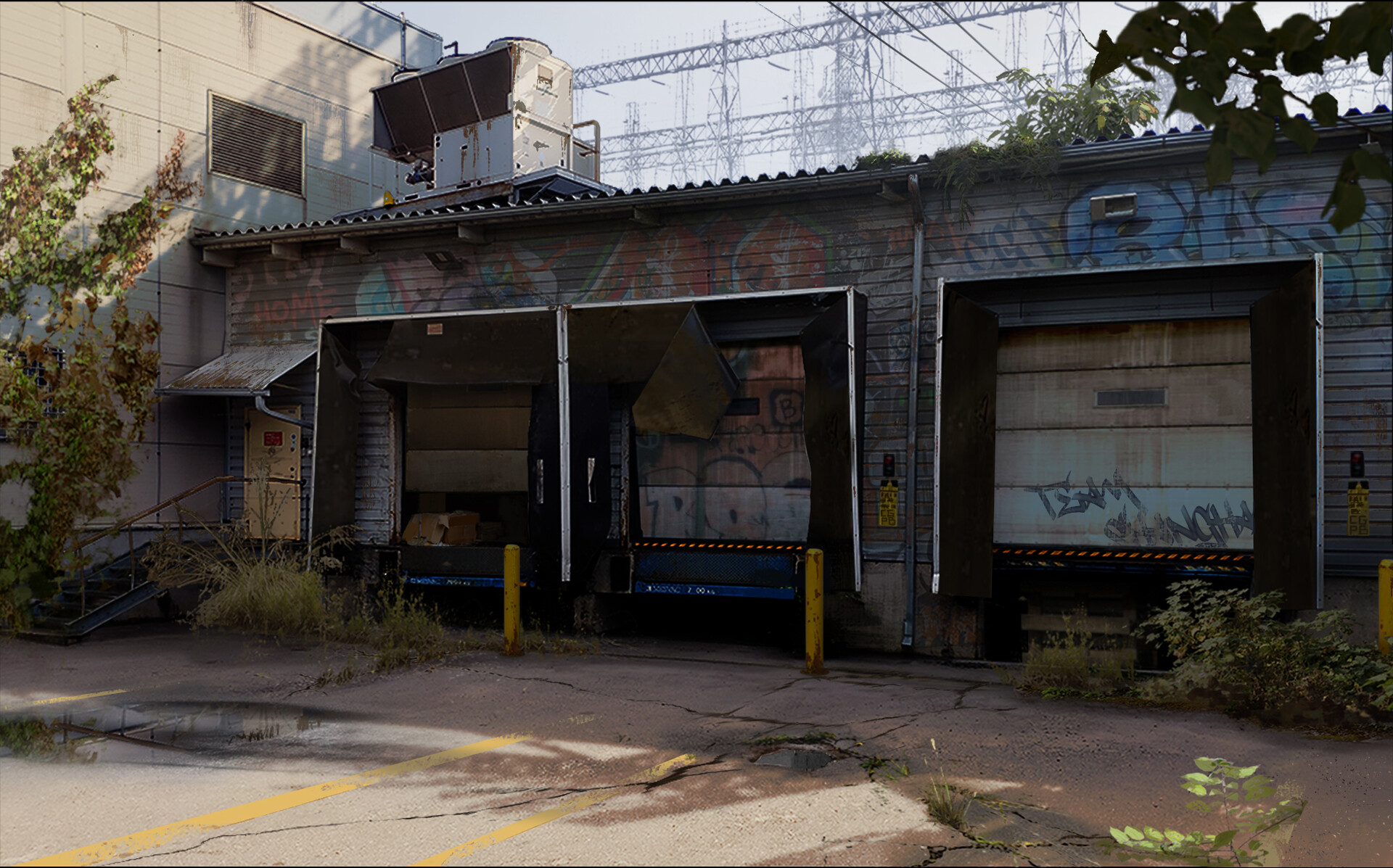The image depicts a seemingly abandoned loading bay at the back of a building on a clear daytime. The structure, with its faded gray siding, is covered in a patchwork of graffiti featuring a mix of blues, reds, purples, and dark grays, although the graffiti appears random and indistinguishable. The three wide vertical rectangular doorways, presumably once used for loading trucks, are trimmed in light gray steel and have doors that roll upwards. The foreground reveals a light gray, cracked, and worn concrete pavement, with patches of green shrubbery and grass sprouting through. There are also signs of rusting white trucks parked nearby, adding to the neglected ambiance. Towards the left, a ramp leads to a teal-colored entrance door under a small awning. Overhead, a light blue sky is visible, punctuated with electrical towers and wires, hinting at a once-busy industrial site now fallen into disrepair.